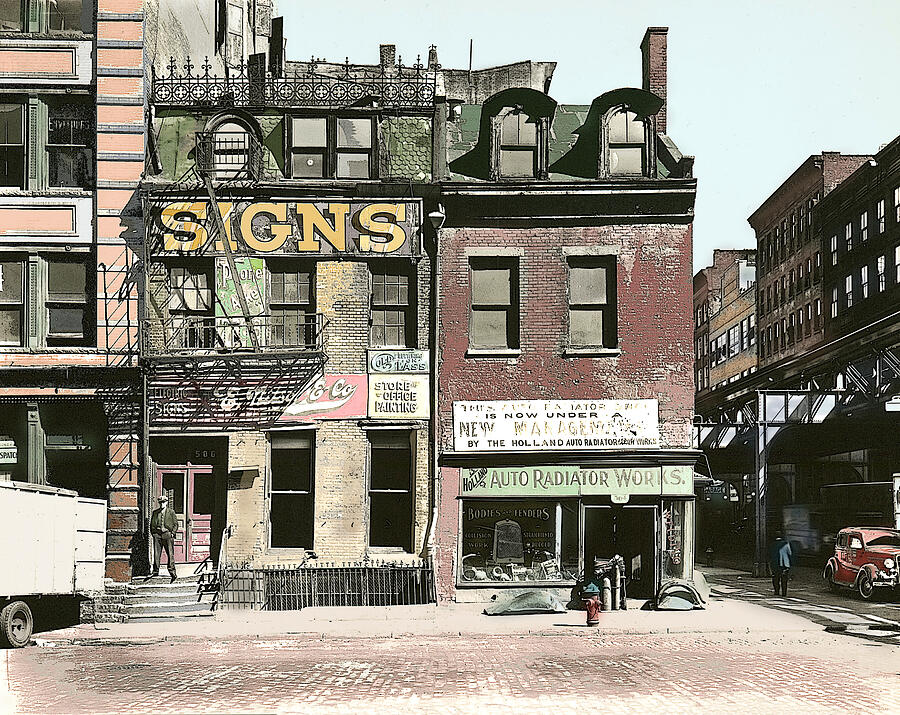This is a vertical rectangular image, likely an artwork rather than a photograph, depicting the front of two side-by-side buildings in an old-timey city setting. The scene is set during the daytime with a light blue sky in the background. The building on the right is three stories tall, constructed of darker red brick with dark green trim, and features a green sign above the first floor reading "Holland Auto Radiator Works." The left building is also three stories tall, made of very weathered light yellow brick with much of its color stripped off. A prominent yellow sign across the second story says "SIG&S Signs." Beneath this sign, there is a fire escape, and just below that, another red sign that is partially legible, mentioning "store office painting." The street in front of the buildings is made of brick, and an old-timey red car is parked to the right. Various other signs, chimneys, and fire escapes add to the historical ambiance, with some text worn and difficult to decipher. Additionally, there is a man standing in a doorway, adding a human element to the scene.